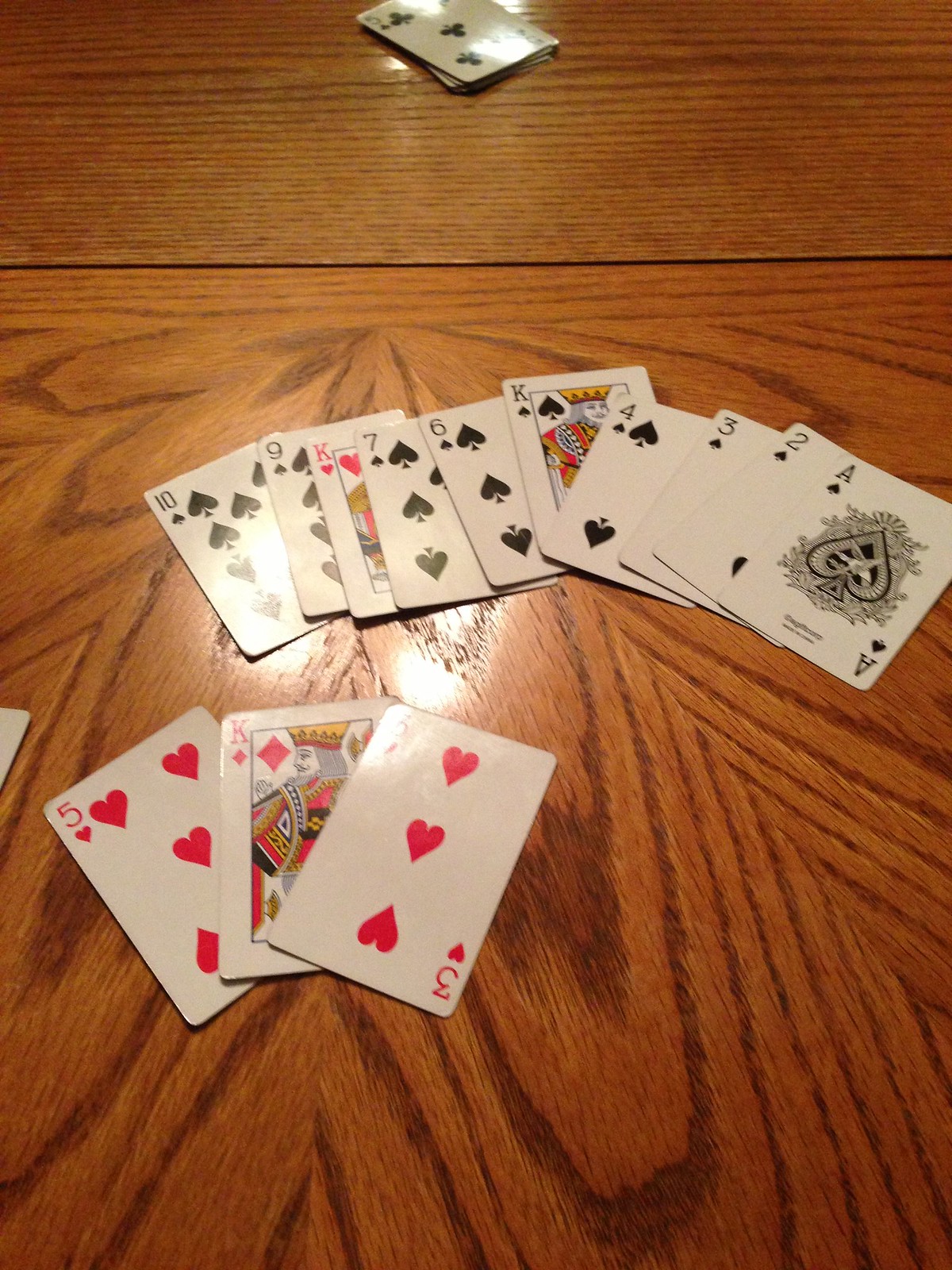The indoor digital photograph showcases two tables pushed together, both exhibiting a brownish tint with darker grain lines running horizontally on the top table. A distinct black line divides the tables, while the bottom one's grain pattern resembles flower petals, adding an aesthetically pleasing touch.

Centrally positioned at the top of the image is a cut deck of playing cards, featuring the five of clubs prominently displayed upright against a white background. Bright white light, seemingly from two different sources, reflects off the cards.

Dominating the main section of the photo is an array of club cards spread out across the scene. Only the corner of a small white card is visible on the left edge, suggesting its smaller size. The top row features a sequence of cards: the ten of clubs, the nine of clubs, the king of hearts, the seven of clubs, the six of clubs, the king of clubs, the four of clubs, the three of clubs, the two of clubs, and the ace of clubs, potentially forming a meaningful sequence.

On the bottom left, the five of hearts and the three of hearts are displayed. Additionally, the king of diamonds, characterized by a yellow crown and a white face looking right, adds a regal touch to the collection with its vibrant red diamonds.